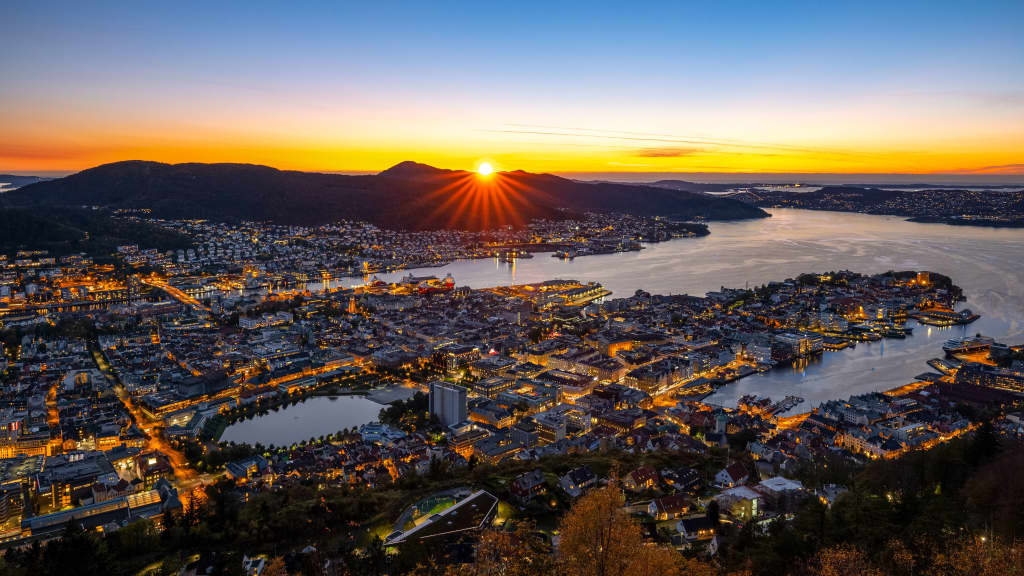The image, captured from an aerial perspective likely by a helicopter or airplane, depicts a populous coastal city bordered by water, possibly a marina or harbor, and surrounded by mountains. The vibrant, HDR-enhanced photo shows the skyline at either sunrise or sunset, with the sun positioned centrally, casting a dramatic silhouette of a mountain against a sky vividly painted in hues of blue, yellow, and orange. The urban landscape below is illuminated by the golden-orange lights of numerous office buildings, apartment complexes, and houses, along with the headlights from the busy traffic on the highways. A notable feature is an inland lake on the left, possibly man-made and not directly connected to the primary body of water. The water itself, a light grayish color, appears to be flowing gently, contributing to the serene yet dynamic atmosphere of the scene.